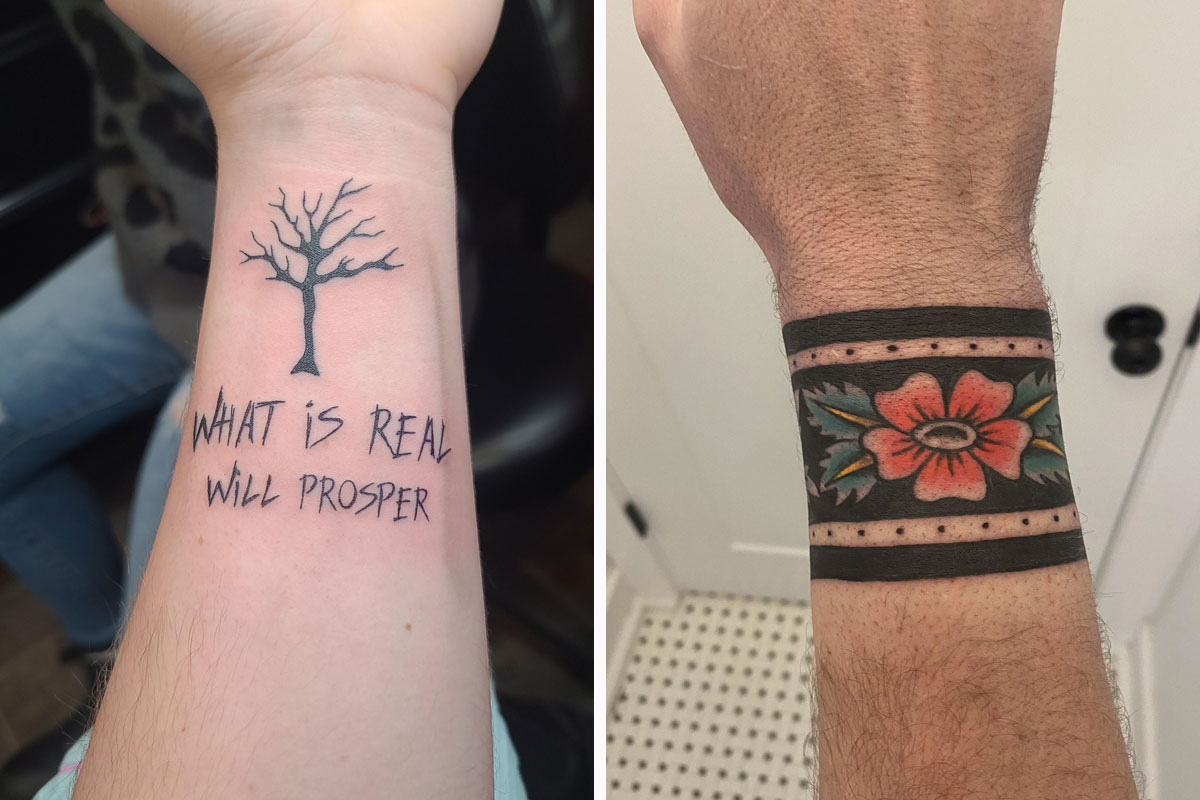The image is a composite of two vertical photographs placed side by side, separated by a vertical white border. The left photograph captures the underside of a man's left forearm and wrist, displaying a fresh tattoo of a leafless black tree and the words “what is real will prosper” beneath it. The skin around the tattoo is red and irritated, indicating it was recently done. In the background, a person dressed in blue jeans and a black and gray top is seated in a black leather chair.

The right photograph shows the back of what is likely a different man’s right wrist, with the forearm extending upwards. This wrist is adorned with a bracelet-like tattoo: two black horizontal bands at the top and bottom, bordered with small white dots, surrounding a central red, pink-tipped flower with two green leaves on each side. The background setting reveals a bathroom with a white door featuring a black doorknob and a vented floor visible at the bottom of the frame.